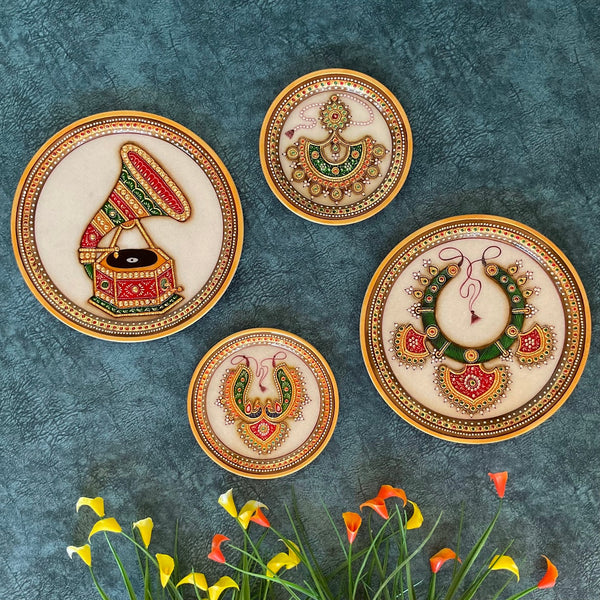The image features an assortment of four intricately designed decorative plates set against a background of varying shades of blue and teal green. The two larger plates are positioned on the left and right side of the image and are adorned with elaborate braided borders. The plate on the left depicts an old-fashioned phonograph with a prominent sound horn, featuring alternating stripes of red, gold, and green. A black record sits on the crimson, gold, and green player. The plate on the right displays a green horseshoe-shaped necklace embellished with yellow circles and three pink and gold bird-shaped pendants.

The two smaller plates—a top one and a bottom one—are similarly bordered with dot-like woven designs. The top one features what resembles a segmented bell-like structure in green, orange, and yellow, with seven round, yellow protrusions. The bottom one also shows a necklace, this time with fewer, single pink and gold bird-shaped pendants.

At the very bottom of the image, green grass is speckled with vibrant yellow and peach-colored flowers, grounding the visually rich and colorful plates above. The overall palette includes shades of blue, green, gold, red, orange, yellow, and peach, yet the image is devoid of any text, numbers, people, or animals.